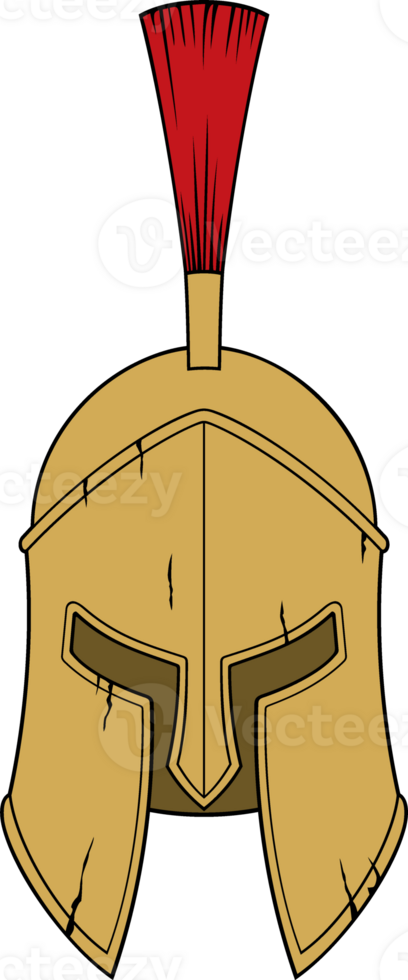The image reveals a stock photo from the website Vecteezy, identifiable by the three watermarks surrounding its logo. It depicts a front-facing Spartan helmet, notable for its substantial battle damage—exhibiting at least nine distinct scratches and cracks throughout its surface. The helmet features a distinctive, pointed nose guard, and its structure is gracefully curved from the top, narrowing towards the center before flaring out around the cheek area. Predominantly gold or bronze in color, the helmet is adorned with an iconic bright red mohawk—resembling a fan or broom—jutting out from the top. Despite the wear and tear, including scars above the eyes and along the middle, the helmet retains a monumental and resilient appearance, reminiscent of the USC Trojan insignia.